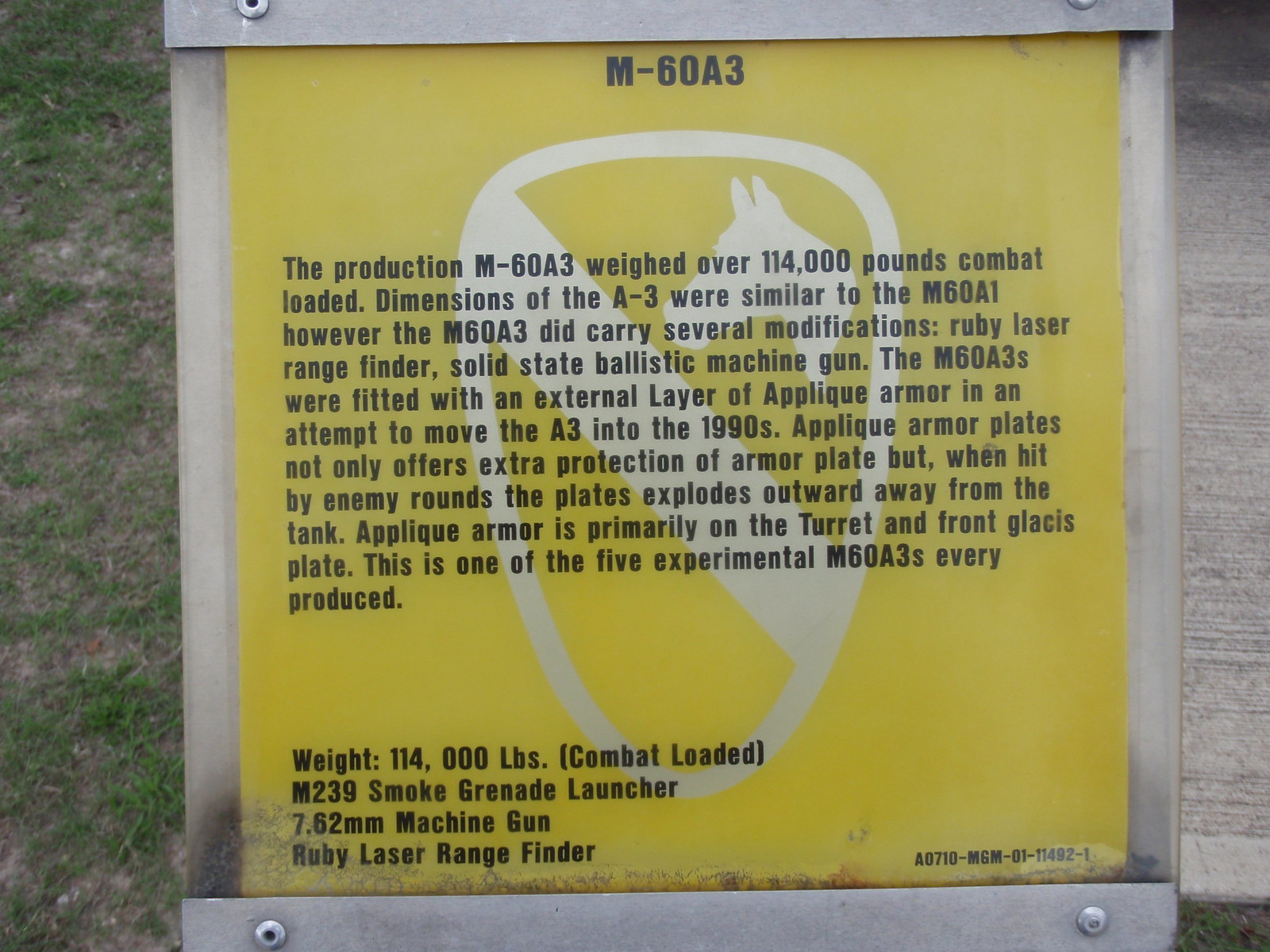The image features a detailed sign set against a background that includes both wood and grass. The sign, surrounded by a thin silver strip, appears to be either paper or plastic and is affixed to a frame positioned outdoors, likely beside a cement road. The sign has a yellow background with black print, with the heading "M-60A3" prominently displayed at the top. Below the heading, a paragraph provides comprehensive information, noting that the M-60A3 tank weighed over 114,000 pounds when combat-loaded. It states that the dimensions are similar to the M-60A1 but highlights several modifications such as a ruby laser rangefinder, solid-state ballistic machine gun, and an external layer of applique armor designed to offer additional protection and adaptability into the 1990s. The sign also notes the presence of a circle with a line through it, featuring a dog's head, indicating it might not be safe for pets in the area. This informative block of text is likely zoomed in to detail something nearby, possibly one of the five experimental M-60A3 tanks ever produced, which were fitted with M-239 smoke grenade launchers and 7.62 millimeter machine guns.